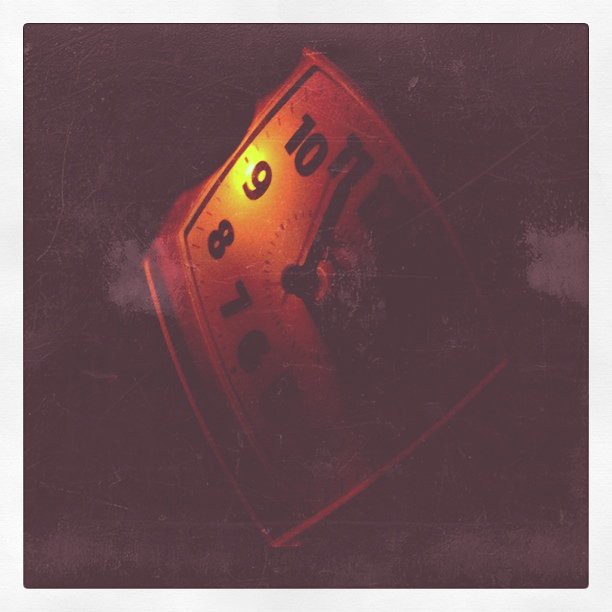This image depicts a very blurry, low-resolution photo of a square-shaped, old-style alarm clock, viewed sideways in a dimly lit, almost completely dark setting. The left side of the clock is partially illuminated, revealing the block numerals 6, 7, 8, 9, 10, and 11, with a small light near the 9 giving an orange-amber glow. The right side of the clock is obscured by heavy shading, making the numbers 12 through 5 almost invisible. The minute hand is faintly visible, pointing towards the 11, while the position of the hour hand remains indiscernible. The background is predominantly black with spotty shades of gray and two barely noticeable faded white spots flanking the clock.